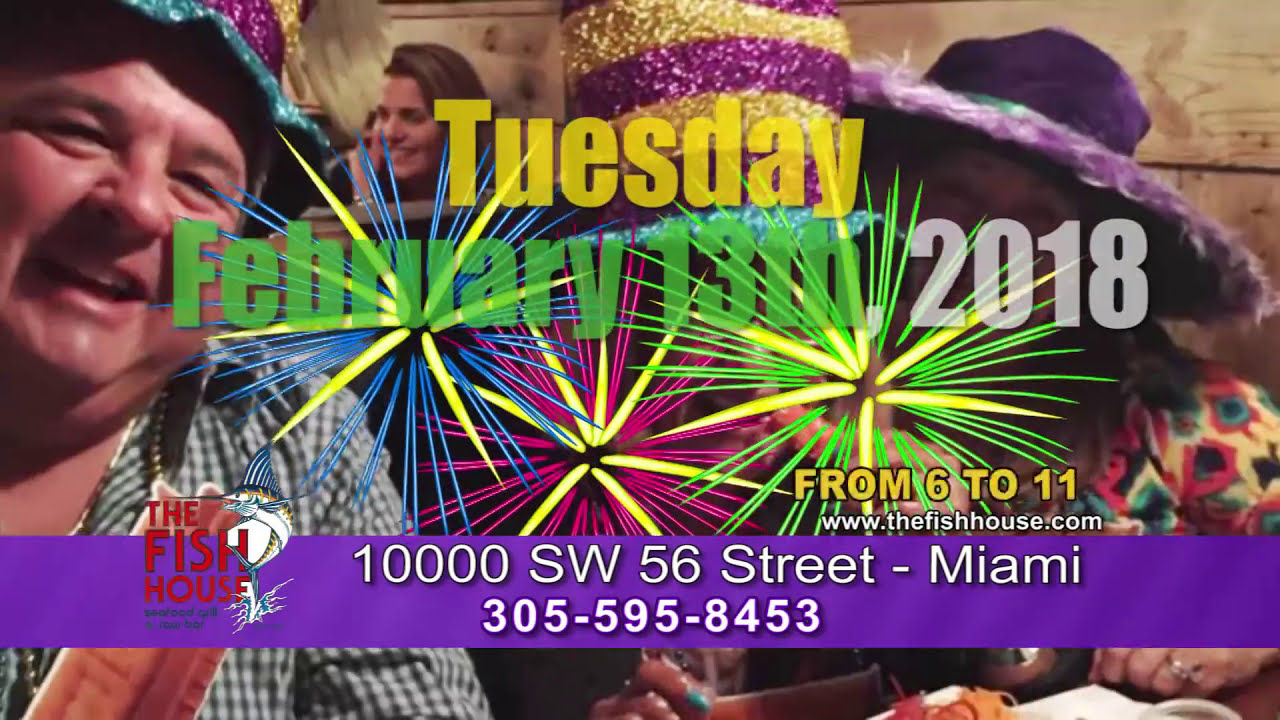The image is an advertisement banner for an event at The Fish House, located at 10,000 Southwest 56th Street, Miami. The banner prominently features a purple section on the bottom displaying the address and phone number, 305-595-8453. The event details, "Tuesday, February 13th, 2018, from 6 to 11," are written in various colors: "Tuesday" in yellow, "February 13th" in green, and "2018" in gray, with the website www.thefishhouse.com included. The background depicts three festively dressed individuals, suggesting a lively and fun atmosphere. These individuals are in party attire with colorful hats; one person in the foreground wears a hat with shiny blue, purple, and gold stripes, and a basic white and gray small checkered plaid shirt. Another person, a female, wears a fuzzy purple hat. Behind them, partially obscured by the banner and decorated with fake firework images, there are more people and a wooden plank wall, enhancing the festive setting.